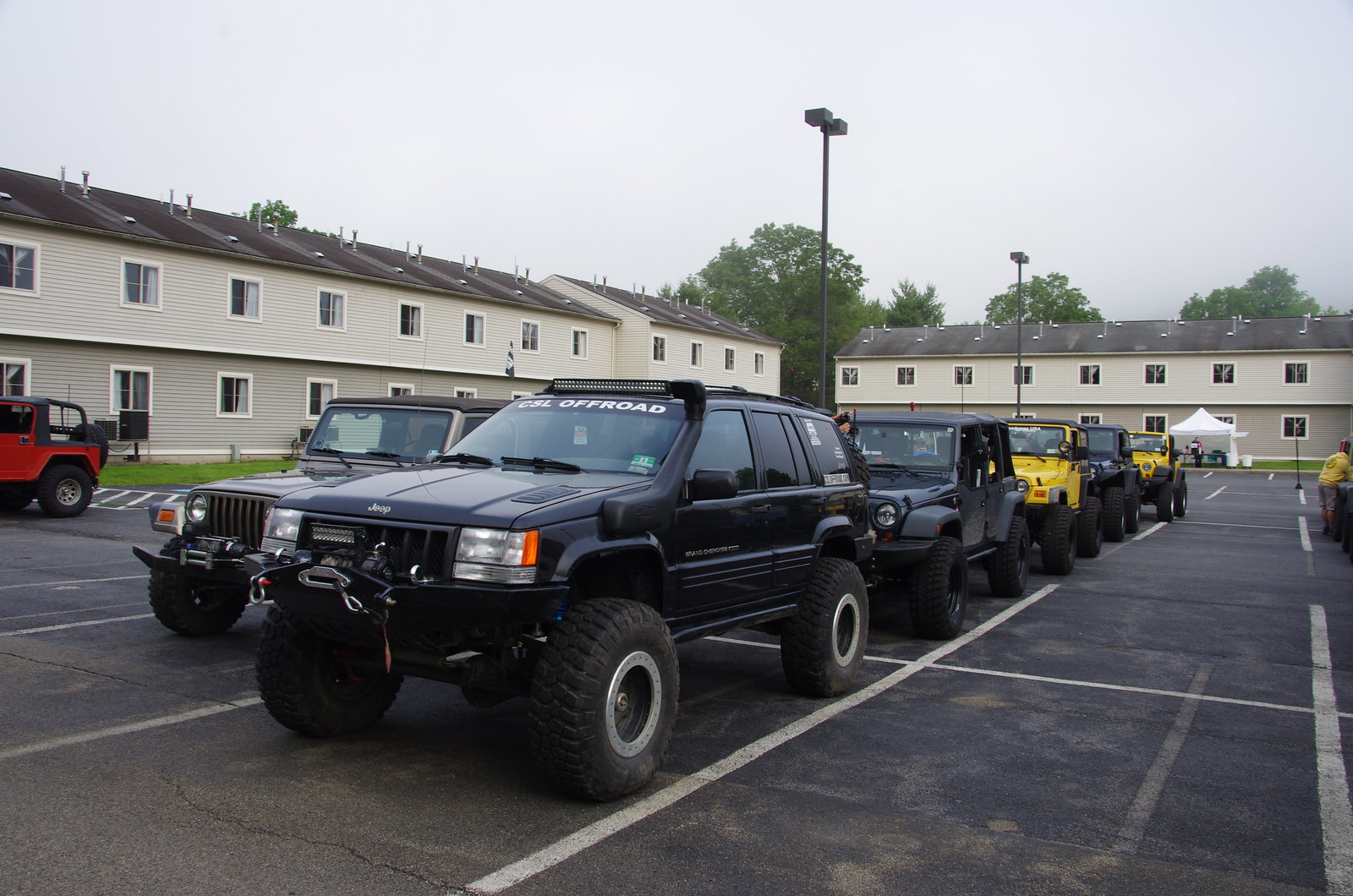The photograph captures a large parking lot filled exclusively with various Jeep vehicles, ranging from classic Jeep Wranglers to Jeep Cherokees, with vibrant colors contrasting against the black pavement and white painted parking lines. The Jeeps, predominantly equipped with lift kits and large off-road black tires, are meticulously arranged in a two-by-two formation, totaling around five or six rows. Notable among the lineup is a black Jeep Cherokee prominently positioned at the front, while "CSL Off-Road" is inscribed on the windshield of another Jeep in the foreground. Toward the back, two yellow Jeeps stand out amidst the predominantly black Jeeps. Adjacent to the rear yellow Jeep, a person in red stands under a white tent. Flanking the parking lot are two-story tan buildings with triangular brown roofs and rows of white-bordered glass windows, which likely serve as apartments. The background further features a bright blue sky on a sunny day and tall, lush green trees.